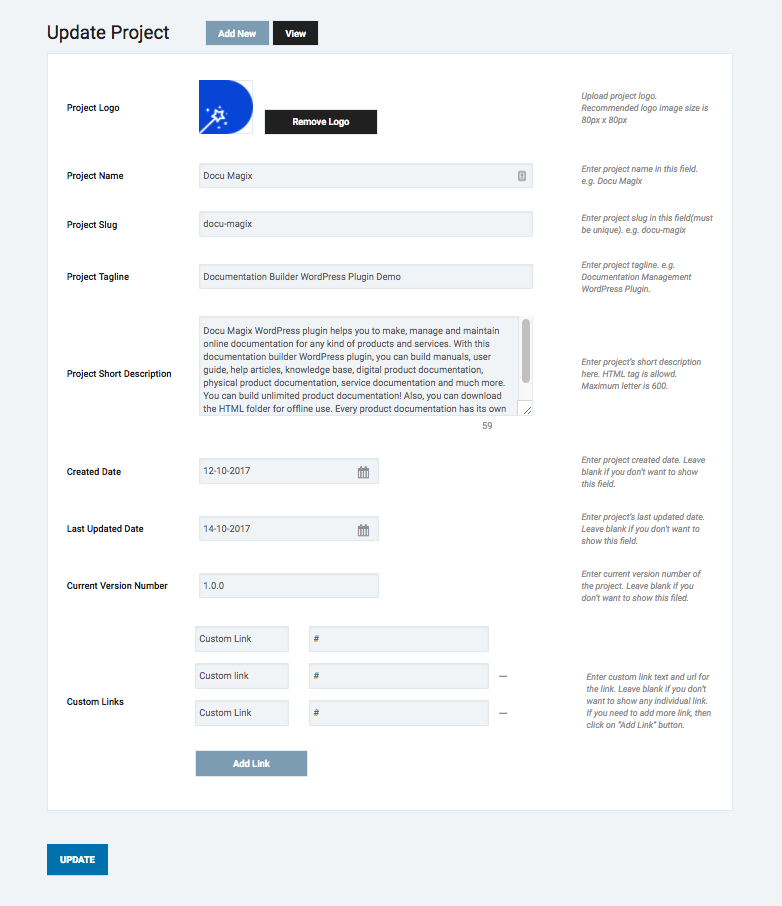The image displays a project update webpage presented in portrait view, suitable for viewing on a tablet or monitor. The webpage is framed with a light blue border and the main content area has a clean white background.

At the top left corner, the heading "Update Project" is prominently displayed. Adjacent to this heading are two buttons: a blue "Add New" button and a black "View" button. The current project being edited is labeled "DocuMagix."

The primary field allows users to enter detailed project information through a series of rows:

1. **Project Logo**: The current logo is already uploaded, with an adjacent "Remove Logo" button providing the option to delete the existing logo and upload a new one.
2. **Project Name**: A text entry box labeled "DocuMagix" is provided for the project's name.
3. **Project Slug**: A row designated for the project's unique identifier.
4. **Project Tagline**: A space for a brief, catchy description of the project.
5. **Project Brief Description**: A larger text box allocated for a short description, complete with a word count indicator at the bottom right corner. The current word count stands at 59 words.
6. **Created Date**: A row for entering the date the project was created.
7. **Last Updated Date**: A row for noting the most recent update date.
8. **Current Version Number**: A section to input the version number of the project.
9. **Custom Links**: Three lines available for entering custom links, with an option to add more links if required.

At the bottom left corner of the border, there is a blue "Update" button, which serves the purpose of saving the current version of the project.